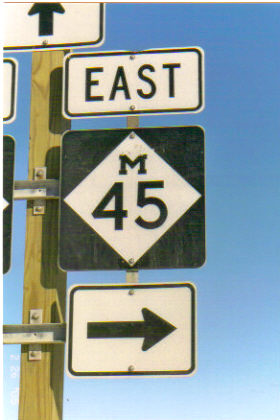This close-up photograph captures a series of street signs affixed to a vertical wooden post, which extends from the bottom to the top of the frame near the left edge of the image. The sky in the background is a clear, vibrant blue, providing a sharp contrast to the signs and wood. At the top of the wooden post, partly visible, is a white sign featuring a bold, black upward-pointing arrow. Directly below it, attached to the right side of the post, is a rectangular white sign with a black border and bold black lettering that reads "EAST." Beneath this is a square black sign with a central white triangle. Within the triangle, the letter "M" is placed at the top, followed by the number "45" in large black text. Further down, there is a square white sign outlined in black, displaying a black arrow pointing to the right.